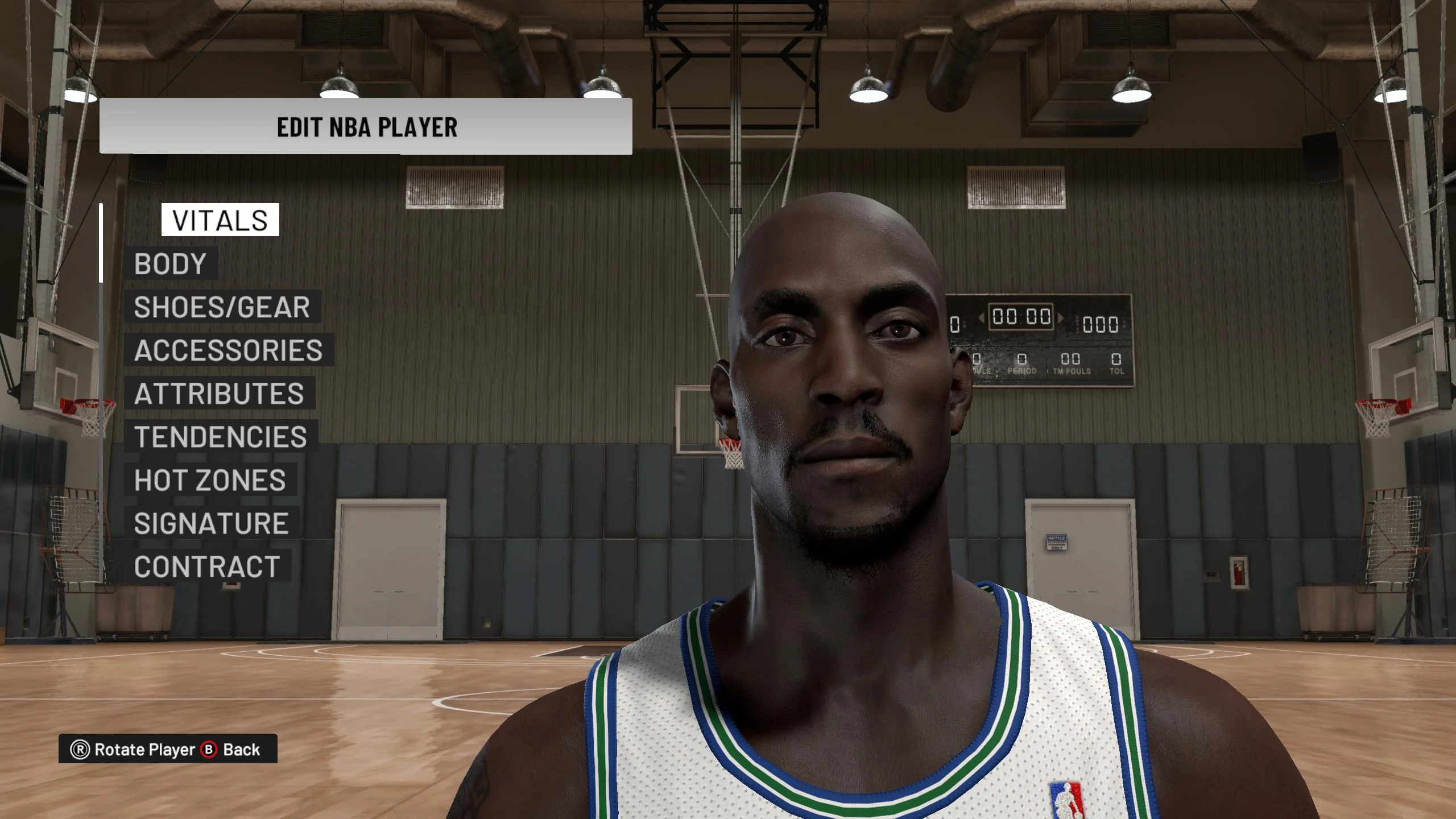This image is a detailed screenshot from a video game depicting an indoor gymnasium setting designed with precision. The background features an expansive gymnasium with fully extended basketball hoops and shiny hardwood floors that reflect their surroundings with a polished gleam. Along the gray, almost black walls, rows of lockers stretch neatly, enhancing the athletic environment. A scoreboard hangs in the distance, and strategically placed lights illuminate the gym floor, creating a realistic ambiance.

In the foreground stands a prominently displayed basketball player. The player is a man with very dark skin, sporting a shaved head and a mustache. He is dressed in a white jersey adorned with green and navy blue stripes around the arms and neckline, signifying team colors. 

To the left side of the screen, a menu titled "Edit NBA Player" lists various customizable options: Vitals, Body, Shoes/Gear, Accessories, Attributes, Tendencies, Hot Zones, Signature, and Contract. 

At the bottom left corner, there is a navigation bar with the option to "Rotate Player" and an additional option to go back, facilitating user interaction within the game's interface. This detailed setup enhances the immersive experience for the player, combining visual and interactive elements seamlessly.